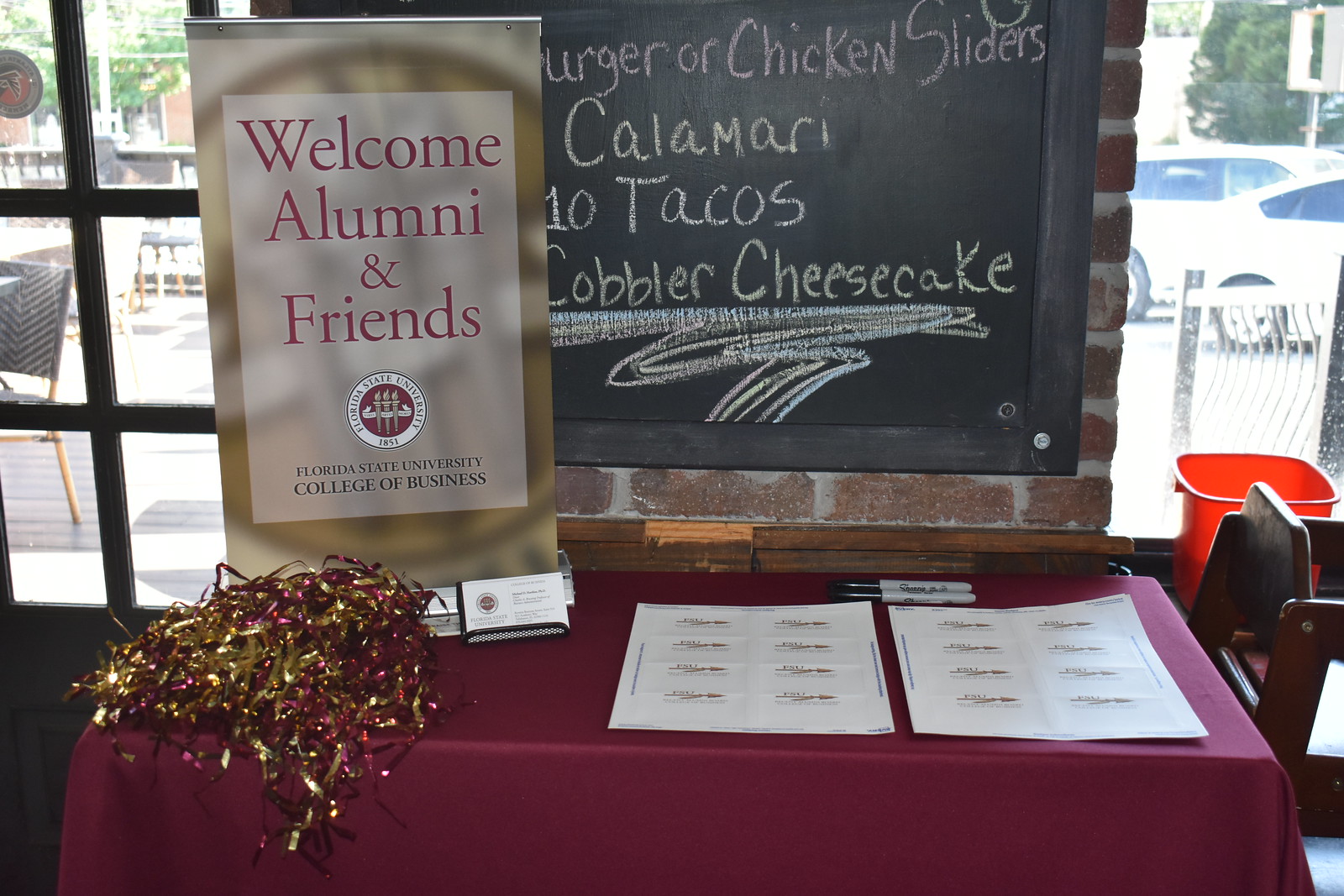This vibrant full-color photograph captures the welcoming ambiance of an indoor alumni event hosted by the Florida State University College of Business. The scene is set in a bright room, well-lit by daylight streaming through large windows that offer a view of an outside parking lot and possibly a patio area. A prominent focal point is a table draped in a maroon tablecloth, positioned against a glass wall. On the table, two Sharpies and sheets of paper intended for name tags are neatly placed, accompanied by a holder filled with business cards. At the forefront, there is a standout sign with gold background and magenta type, reading, "Welcome Alumni and Friends from the Florida State University College of Business," adorned with the university's seal above. In the background, a chalkboard menu lists the food offerings: burgers or chicken sliders, calamari, ten tacos, cobbler, and cheesecake. The event space is also decorated in the university's maroon and gold colors, with additional festive touches like pom-poms or beads adding to the celebratory atmosphere. It appears to be a well-organized gathering spot for alumni, equipped with all the necessities for a welcoming and convivial reunion.